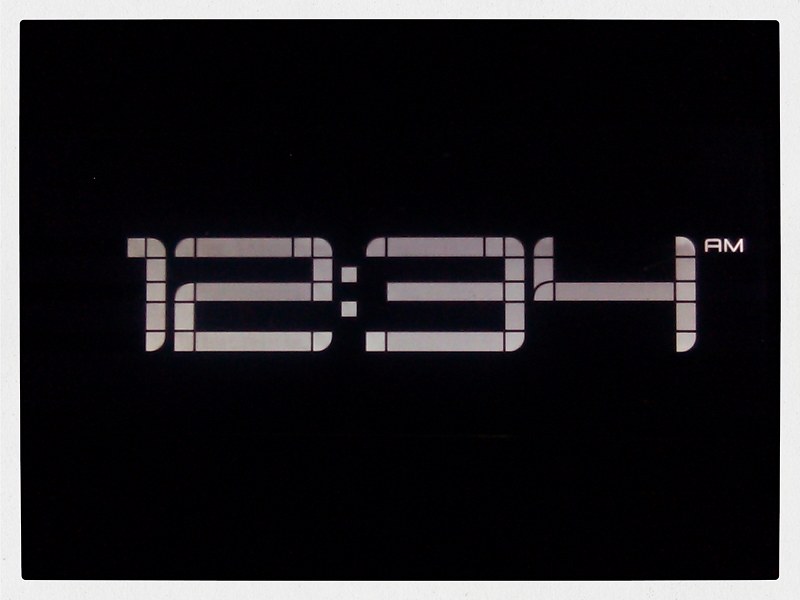This close-up image captures the digital display of a clock reading "12:34 AM" against a solid black background. The white numbers are formed by small rectangular blocks, common in digital time displays. The digit "1" at the front has a distinctive design, with the top end of the "1" slanting to the left and its base featuring a rounded edge. The display is free from any surrounding elements, focusing solely on the time representation.